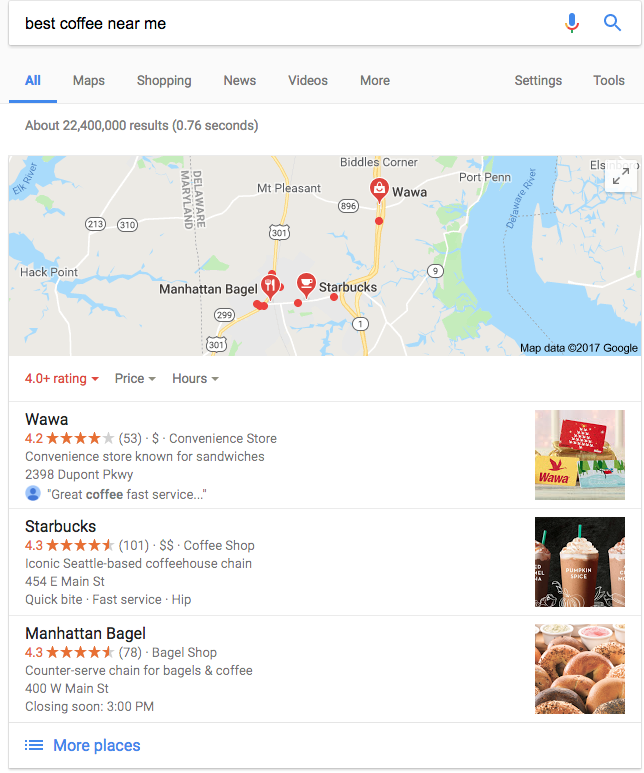The image captures a search results page with the query "best coffee near me" typed into the search bar at the top. Immediately below this, the word "All" is underlined, indicating selected search results, while nearby options include Maps, Shopping, News, Videos, More, Settings, and Tools. The page reports approximately 22,400,000 results found in 0.76 seconds.

A prominent map is displayed below this information, showing the border between Delaware and Maryland. Key locations such as Mount Pleasant, Port Penn, and Hack Point are marked on the map. Red markers indicate various establishments, including Wawa, Starbucks, and Manhattan Bagel. 

Beneath the map, detailed listings begin with:

1. **Wawa** - Rated 4.2 stars, characterized as a convenience store with an emphasis on sandwiches. Located at 2398 Dupont Parkway, its service is described with the phrase "great coffee, fast service." An image on the far right shows the Wawa logo.
  
2. **Starbucks** - Rated 4.3 stars with a double-dollar sign ($$) indicating its price range. This iconic Seattle-based coffee house chain is at 454 East Main Street and is noted for being a quick bite with fast service and a hip ambiance. The accompanying picture on the far right features a close-up of a Starbucks cup labeled "pumpkin spice."

3. **Manhattan Bagel** - Also rated 4.3 stars, this bagel shop offers counter service for bagels and coffee. It is situated at 400 West Main Street and is noted to be closing soon at 3 p.m. The associated image on the far right showcases an assortment of donuts.

This thorough depiction provides comprehensive details for each location, aiding in deciding on the best coffee experience nearby.